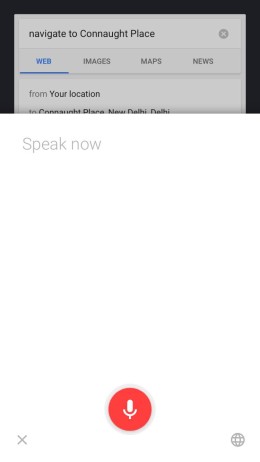This screenshot depicts a Google Maps navigation interface showing a search query for "Navigate to Connaught Place." The user appears to have clicked on the web section, which shows the route from their current location to Connaught Place in New Delhi, India. The screen displays truncated text indicating directions, with a prompt that says "Speak Now" in grey lettering, though it's somewhat faint against the light mode background. 

Overlaying the interface are navigational options visible under Google Images, Maps, and News tabs. At the bottom center, a red microphone button is displayed, alongside a globe icon and an X button, suggesting options for voice input. Notably, the screen is shown within a darker interface, contrasting sharply with the light mode of Google Maps. The purpose of the voice recording or speaking feature in this context remains unclear.